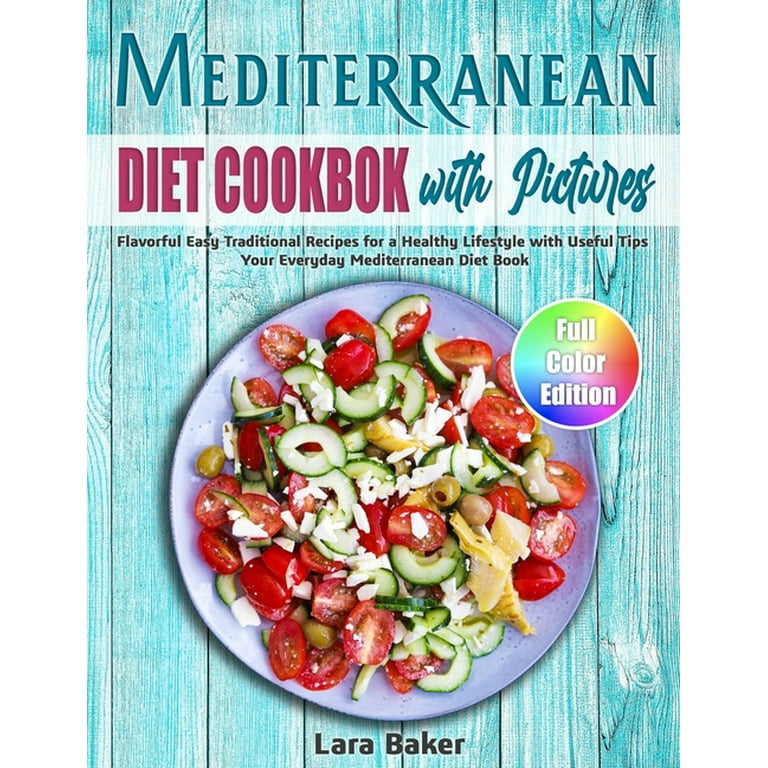The front cover of this Mediterranean diet cookbook, titled "Mediterranean Diet Cookbook with Pictures," features the author's name, Lara Baker, at the bottom. The backdrop depicts a light turquoise, wooden-paneled surface resembling a picnic-style table. At the top of the cover, the word "Mediterranean" stands out in bold blue font, with "Diet Cookbook" erroneously spelled as "Diet Cookboch" in a dark pink color below it. Accompanying this, the phrase "With Pictures" is written in the same blue font, but in italics.

Beneath these titles, a white rectangle contains the subtitle: "Flavorful easy traditional recipes for a healthy lifestyle with useful tips your everyday Mediterranean diet book," all written in small black font. Below this descriptive text, there is a tantalizing image of a Mediterranean salad on a purple circular plate. The salad comprises an assortment of vegetables, including greens, cucumbers, and peppers, alongside olives and cubes of cheese, topped with avocado and tomatoes. Beside this plate, a colorful circular badge reads "Full Color Edition" in white font, emphasizing the vibrant, visual appeal of the cookbook. The author's name, Lara Baker, is prominently placed at the bottom of the cover in black font.